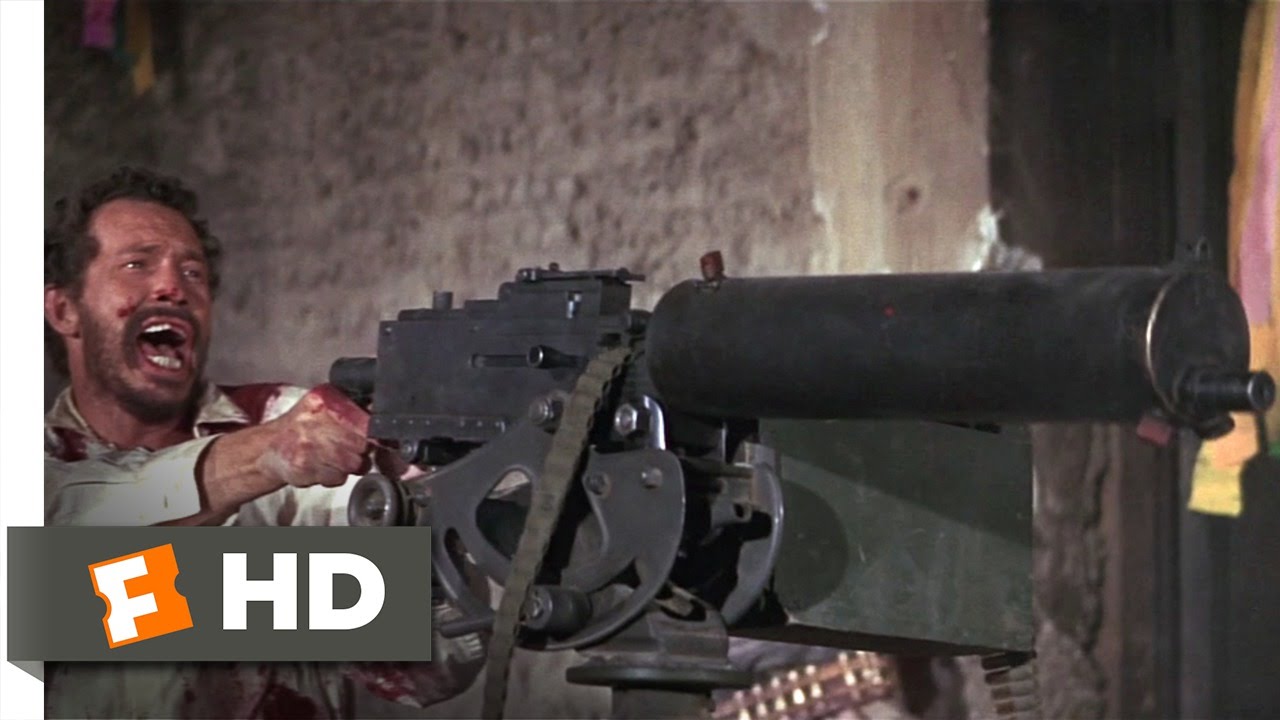This is a rectangular, horizontal color photograph that appears to be a still from an old movie, likely advertising Fandango's HD service given the logo in the lower left corner, featuring a white "F" on an orange block next to "HD" in white. The scene depicts a bearded man with curly dark hair and khaki attire, standing in a decrepit, burnt-out building with a brick wall and a partially visible door with a curtain. He is in an intense and violent moment, his mouth wide open as if screaming, with some blood on his face, firing a large, belt-fed machine gun or Gatling gun. The atmosphere and setting suggest a sense of historic conflict, potentially from a Hollywood western or an old war movie, bringing to mind the gritty intensity of a Clint Eastwood spaghetti western. The lifelike detail and dramatic action contribute to the photograph's gripping and violent nature.